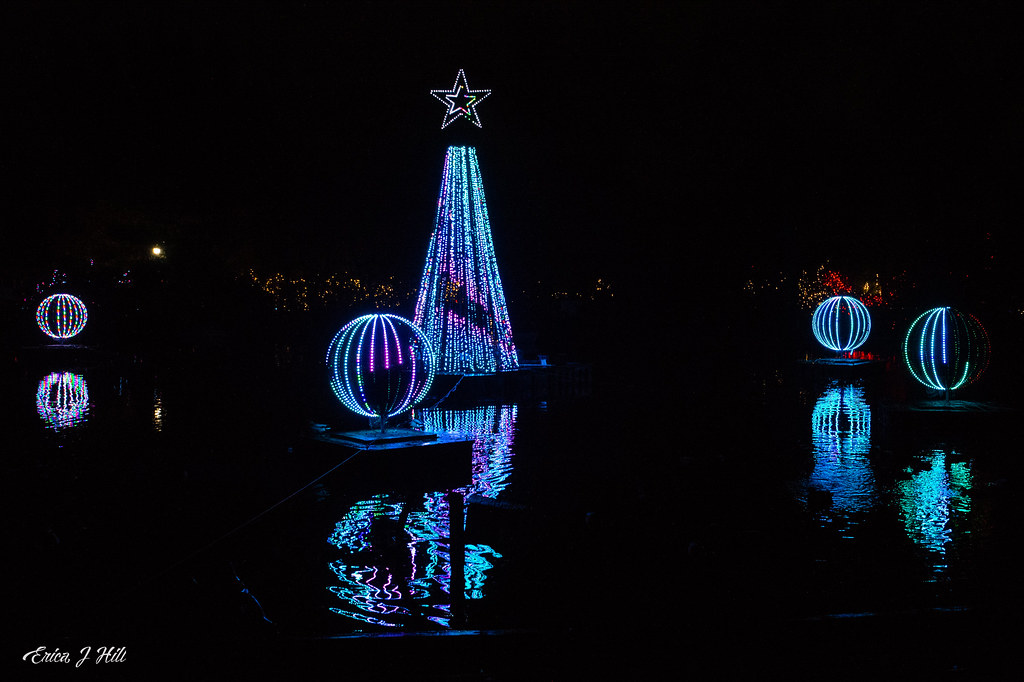In this captivating nighttime photograph, the serene darkness is illuminated by a mesmerizing display of Christmas-style lights over a body of water. Central to the scene, a cone-shaped formation reminiscent of a festive tree ascends with a gradient of teal, pink, and blue hues, culminating in a neon star. The foreground features a multicolored orb imbued with white, green, and red lights, casting vibrant reflections on the dark water surface. Additional spherical lights are arranged across the scene: a glowing orb sits on a platform near the center while towards the right, bluish-purple LED-lit orbs add to the dreamlike ambiance. The image is signed "Erica J. Hill" in cursive on the bottom left corner, subtly anchoring this enchanting spectacle. Distant, faint lights suggest the presence of buildings, further enriching the backdrop of this immersive light show.